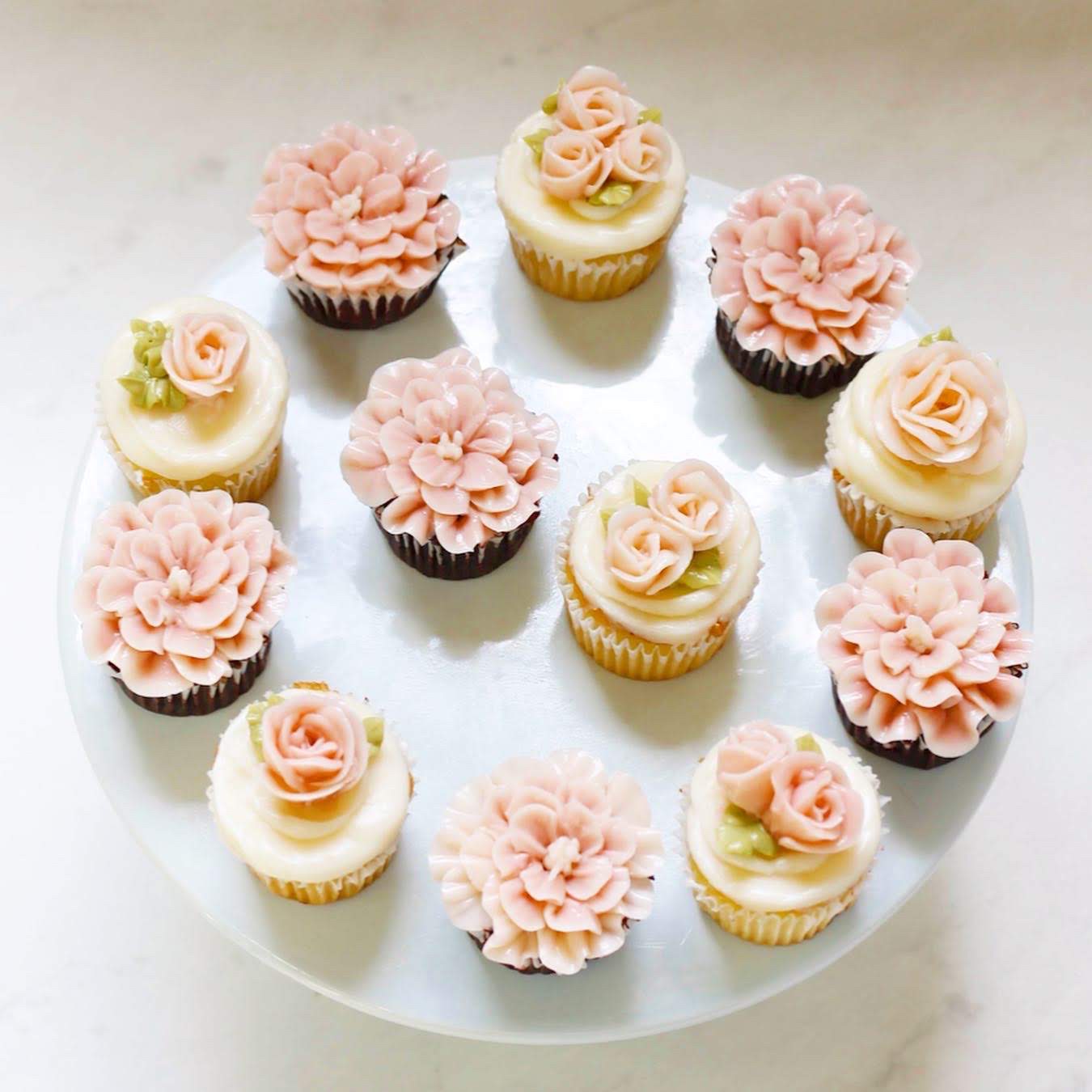A round marble cake stand adorned with an array of delectable cupcakes sits gracefully on a pristine white marble countertop. The elegant cake stand, also crafted from white marble, perfectly complements the countertop, creating a seamless and sophisticated backdrop. On the cake stand, a delightful assortment of cupcakes is arranged, showcasing both chocolate and vanilla varieties. Each cupcake is meticulously decorated with either white or pink icing. The vanilla cupcakes feature delicate pink roses on top, adding a touch of elegance, while the chocolate cupcakes boast larger, more elaborate pink flowers that generously cover the entire surface of the cupcake. This exquisite display of cupcakes not only promises delicious flavor but also delights the eye with its artistic presentation.